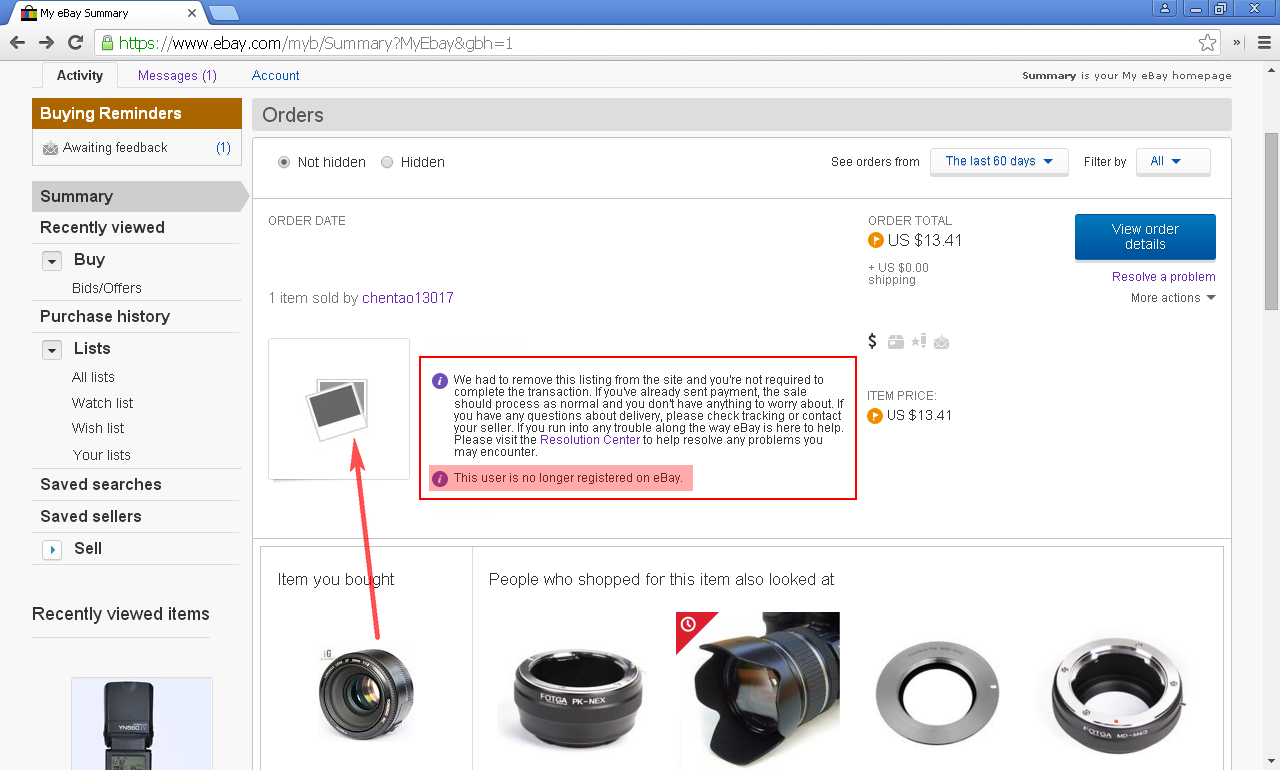The image showcases a screenshot of an eBay website, specifically the Activity tab of a user's account. In the browser's search bar, the URL "www.ebay.com" is faintly visible. The top navigation bar displays three tabs: "Activity," "Messages" (with a notification badge showing the number 1), and "Account," with the current view set on the "Activity" tab.

Below the navigation tabs, the page offers various sections. The primary section starts with "Buying Reminders," followed by a nested list structure. First is "Summary" and "Recently Viewed," which is slightly indented. Under "Recently Viewed," the "Buy" category appears, leading to a bold "Purchase History." Beneath "Purchase History," another indented list includes "List," featuring subsections "All Items," "Search Lists," and "Watch Lists."

Additionally, bold headings like "Save Searches" and "Save Sellers" are present. "Save Sellers" expands into an indented "Sell" category. The section concludes with "Recently Viewed Items," showing a photo of what appears to be a camera lens, indicating the user's browsing interest.

In the center of the page, there is a section titled "Orders," displaying some difficult-to-read buttons and other elements like "Order Date" and images representing various camera lenses and equipment.